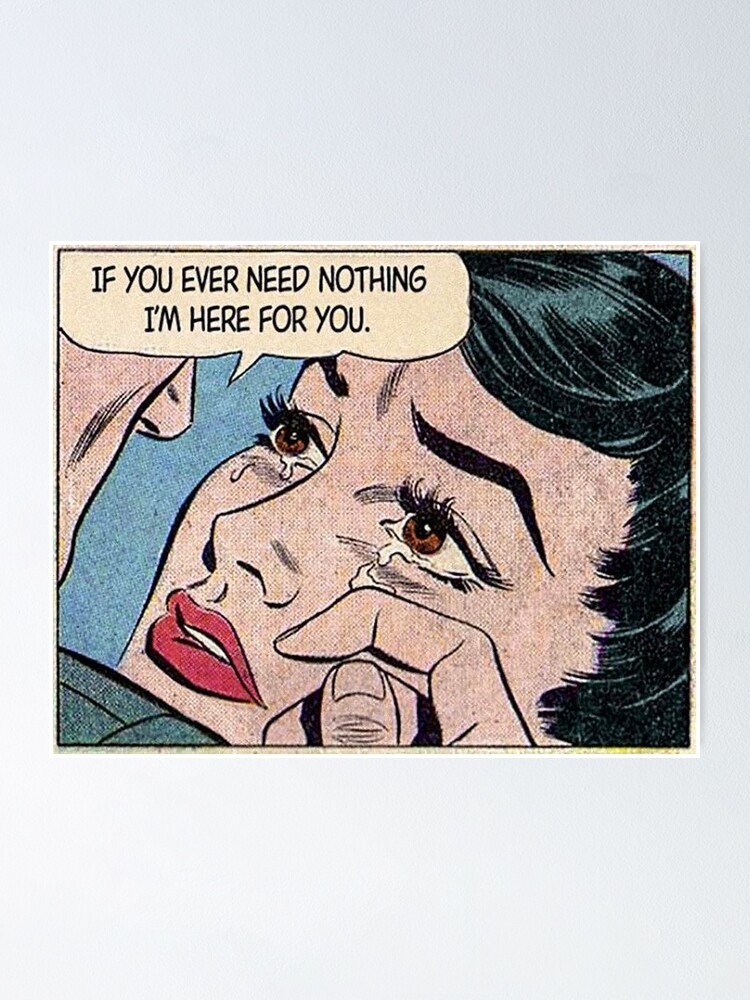In this vintage comic book panel reminiscent of classic pop art, a tender moment unfolds between two characters. A woman with black wavy hair, brown eyes, long eyelashes, and red lipstick dominates the frame. Her tear-streaked face reflects her emotional state as she looks up at a man gently wiping away her tears with his thumb and finger. The man, only partially visible, reveals just the side of his face and the shoulder of his green felt-patterned suit. The dialogue bubble captures his comforting words, "If you ever need nothing, I'm here for you." The bold hand-brushed black lines and simple flat colors against a textured newsprint background further accentuate the emotional depth of this intimate scene.